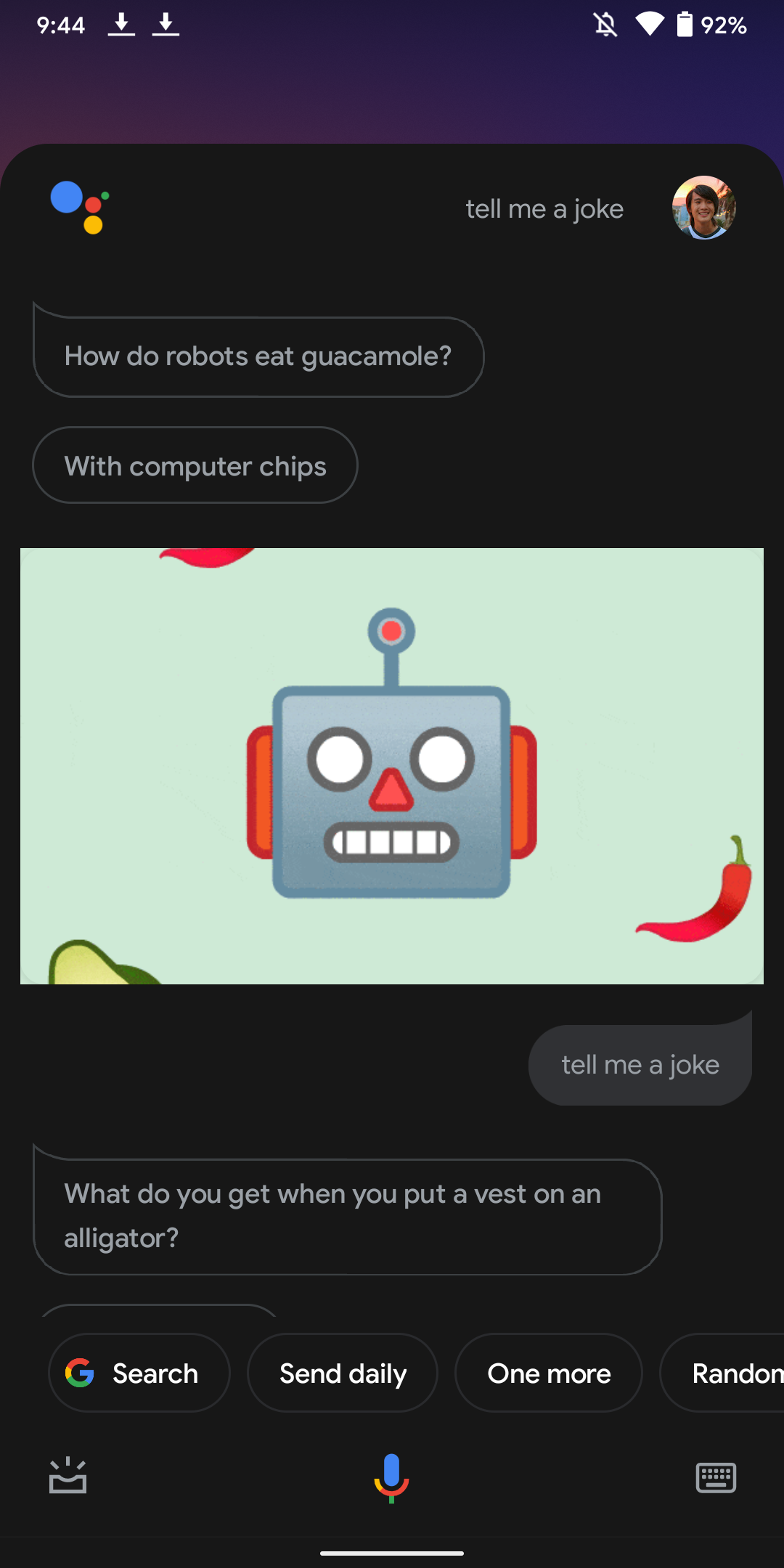The image appears to be a screenshot from an Android smartphone, showing a Google Assistant interaction. At the top, the status bar indicates it is 9:44, with the battery at 92%, sound notifications on, and active download notifications. The user has typed "tell me a joke" into the search bar of the Google Assistant, identifiable by a user avatar in a circle. The Assistant replies with the joke, "How do robots eat guacamole? With computer chips," accompanied by an image of a robot head and a red chili pepper on a mint green background. The user repeats the request, prompting the Assistant to ask, "What do you get when you put a vest on an alligator?" Although the punchline is not visible. Below this exchange, there are options labeled Google Search, Send Daily, One More, and Random, along with microphone and keyboard icons. At the top of the smartphone screen, standard indicators for time, downloads, wireless signal, and battery state can be seen.